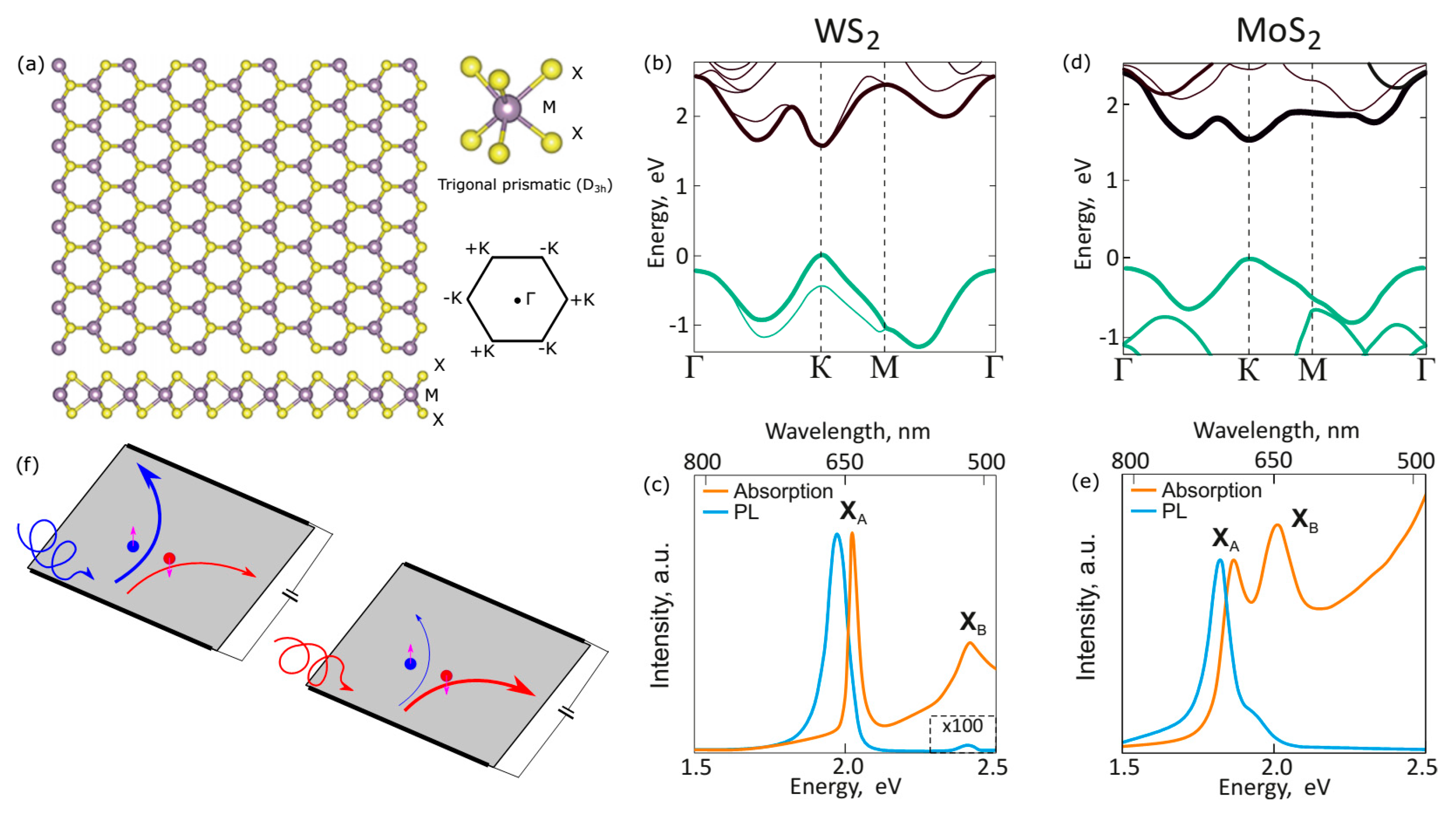The image is a complex diagram likely taken from a chemistry or physics textbook, displaying a series of interconnected graphs and visual data on a white background. In the top left corner, labeled 'A', there is a latticework of blue and red stars connected in a pattern. Below it, there are two diagrams of flat sheets, each with blue and red lines and arrows, alongside several other geometric shapes, such as a trigonal prismatic labeled 'd3h' and another shape surrounded by the labels K+, K, and -K.

Adjacent to this, four graphs are arranged in a grid format, showcasing data related to energy and wavelength for WS2 and MOS2 materials. The top-left graph is labeled "WS2" with the y-axis indicating energy (eV) and features wavy lines colored black and turquoise. Similarly, the top-right graph is labeled "MOS2" with energy (eV) on the y-axis and also features black and turquoise wavy lines. The bottom-left graph denotes wavelength (nm) and intensity (AU) with distinctive peaks represented by turquoise and gold lines. The bottom-right graph also shows wavelength (nm) against intensity (AU), with turquoise and gold lines peaking at different intervals and intensities. 

Overall, the details across the diagrams and graphs seem to depict various properties and behaviors of materials under different conditions, possibly from experimental data concerning energy levels and wavelength intensities.